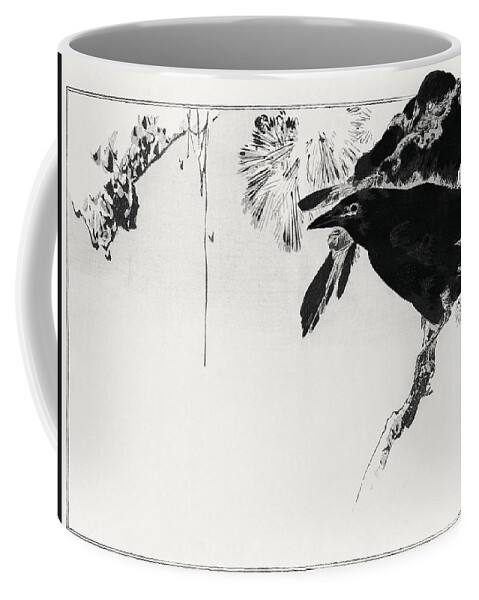A monochromatic photograph captures a distinctive, white coffee mug adorned with a black and white design. The mug itself is slightly taller than average and features a cylindrical shape with a standard handle. The handle is elongated and uniformly curved, extending from just below the rim to near the base.

The design on the mug is intriguing and intricate, depicting a humanoid figure with a wolflike face. This character appears to be wearing a dark, fur-lined cape, which envelops them in a dramatic fashion. Interestingly, instead of traditional legs and feet, the figure seems to have feathers on one side and an ambiguous shape that might be a foot on the other.

Surrounding the figure is a dynamic background, suggesting movement or action. An explosion-like effect is prominently displayed near the character, accompanied by an element that resembles dripping liquid. Additionally, a portion of the background design appears to be melting, adding to the overall surreal and captivating imagery.